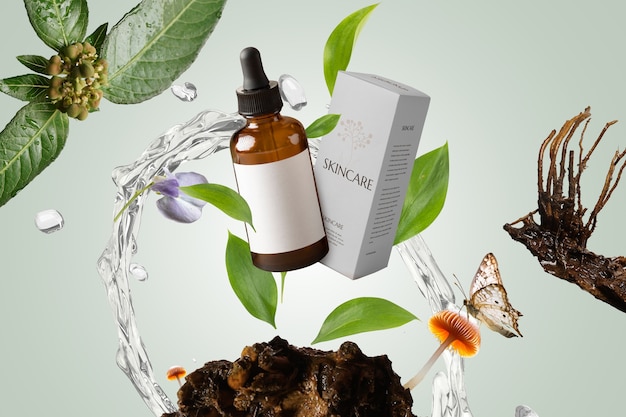The image is a heavily edited product photo featuring a generic brown bottle with a rubber-capped dropper top, lacking any label. The bottle is positioned in front of a plain gray box labeled "skincare." Surrounding the product, various green leaves float around, and a splash of water arches in a crescent shape behind the bottle. The background transitions from a light white center to a darker green towards the edges. At the bottom, a mound decorated with orange and white mushrooms is visible, with a butterfly with white wings perched on one of the mushrooms.